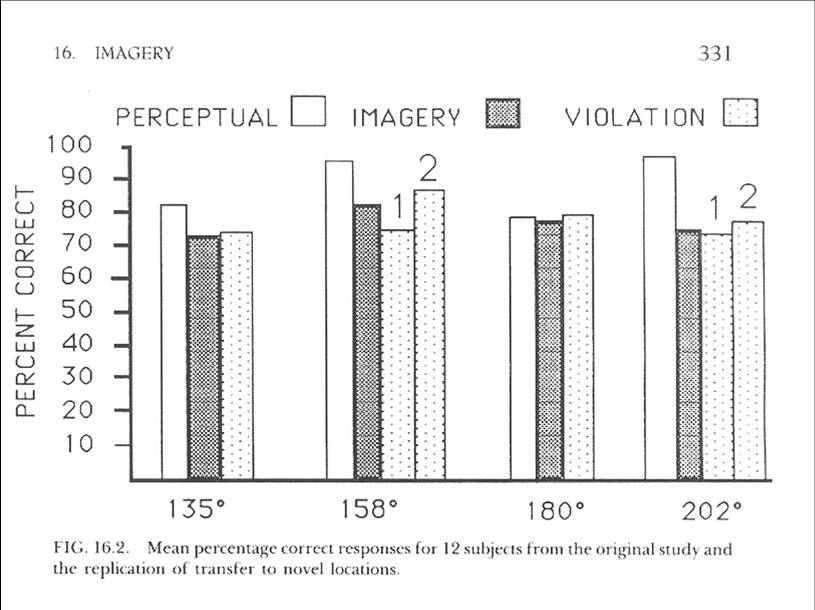The image is a detailed black-and-white page from a book, featuring a bar chart that visually represents data. At the top of the page, the background is white and displays the number 16 in smaller letters and the number 331 in a slightly larger font on the right. Beneath these numbers, the central focus is a bar chart titled "Perceptual Imagery and Violation" which uses different keys: a white box, a gray box, and a polka-dotted box to differentiate categories.

The chart itself shows corresponding bars with varying heights, which are explained on the left side where the vertical axis is labeled "Percent Correct," ranging from 10% to 100%. Horizontally along the bottom, different degrees are marked. Below the chart, a caption reads "Figure 16.2 Mean Percentage Correct Responses for 12 Subjects from the Original Study and the Replication of Transfer to Novel Locations," indicating the results of a study comparing perceptual, imagery, and violation across four degrees: 135, 158, 180, and 202. The data points suggest a range of results, with percentages mostly clustering between 70% and a little over 90%, showing that for these conditions and degrees, the responses were fairly consistent among participants.